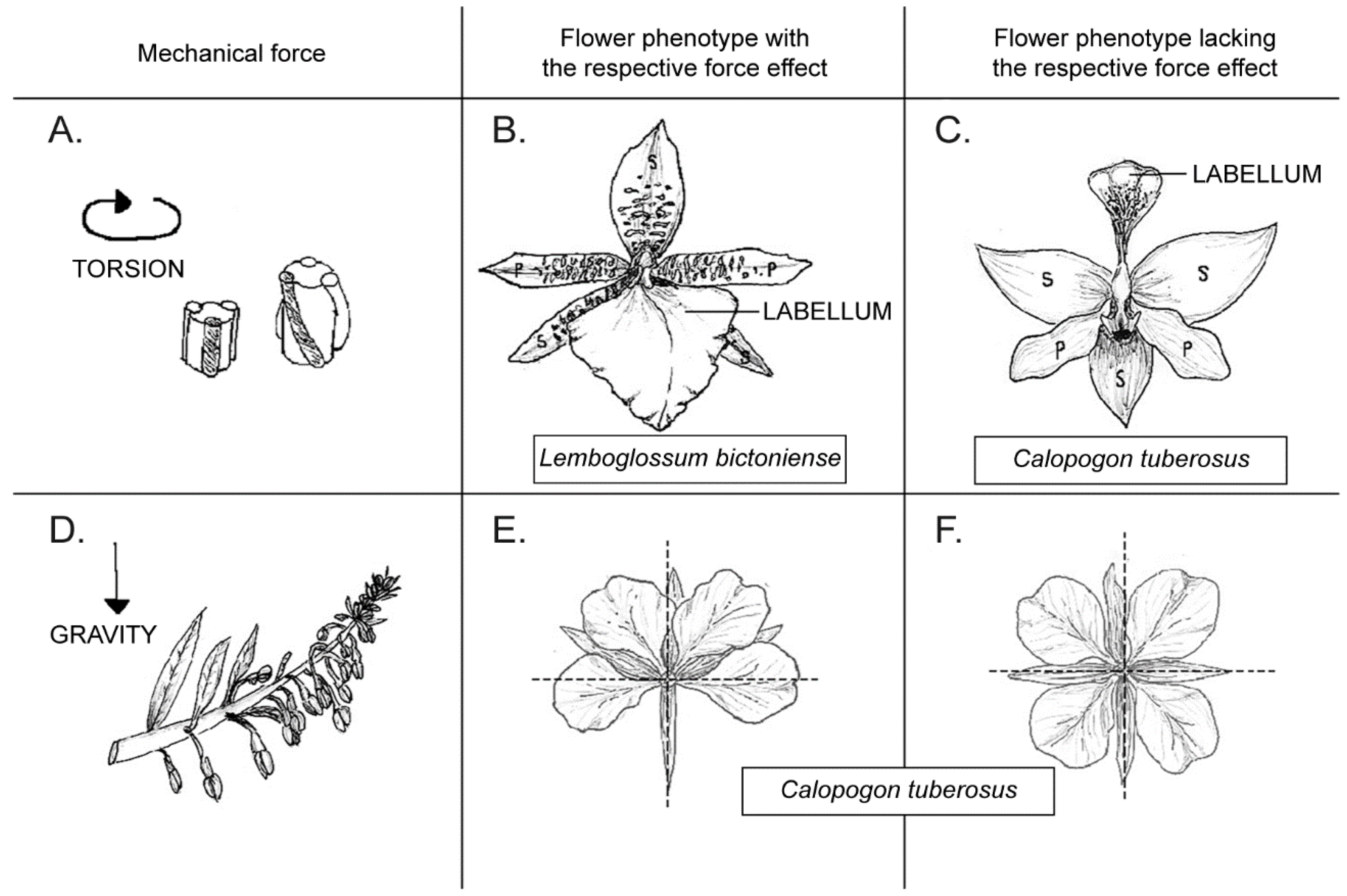The image is a detailed black and white diagram illustrating various flowers and plants, meticulously drawn with what appears to be black ink or marker. The diagram is organized into three columns and two rows, effectively comparing the effects of mechanical forces on flower phenotypes.

In the first column, titled "Mechanical Force," specific forces such as torsion and gravity are depicted. Directly across from each force in the second column, labeled "Flower Phenotype with the Respective Force Effect," are illustrations showing how each force affects the plant's growth. The third column, labeled "Flower Phenotype Lacking the Respective Force Effect," compares these phenotypes by showing plants without the influence of the mechanical forces.

Each section within the grid is labeled from A to F:
- In section A, the mechanical force is "torsion," illustrated by a cylindrical object and an arrow indicating rotational force.
- Sections B and C continue to illustrate various plant forms and their response to torsion, specifically showcasing species like Labellum or Lamoglossum victorinensis and Calopogon tuberosus.
- Sections D, E, and F focus on the effects of gravity, with examples such as flowers that hang downward from a stalk or are divided into quadrants, also including species like Calopogon tuberosus.

The diagram’s meticulous organization and rich details highlight the diverse responses of plant phenotypes to mechanical forces, providing a comparative visual study of the influence these forces exert on plant structure and form.